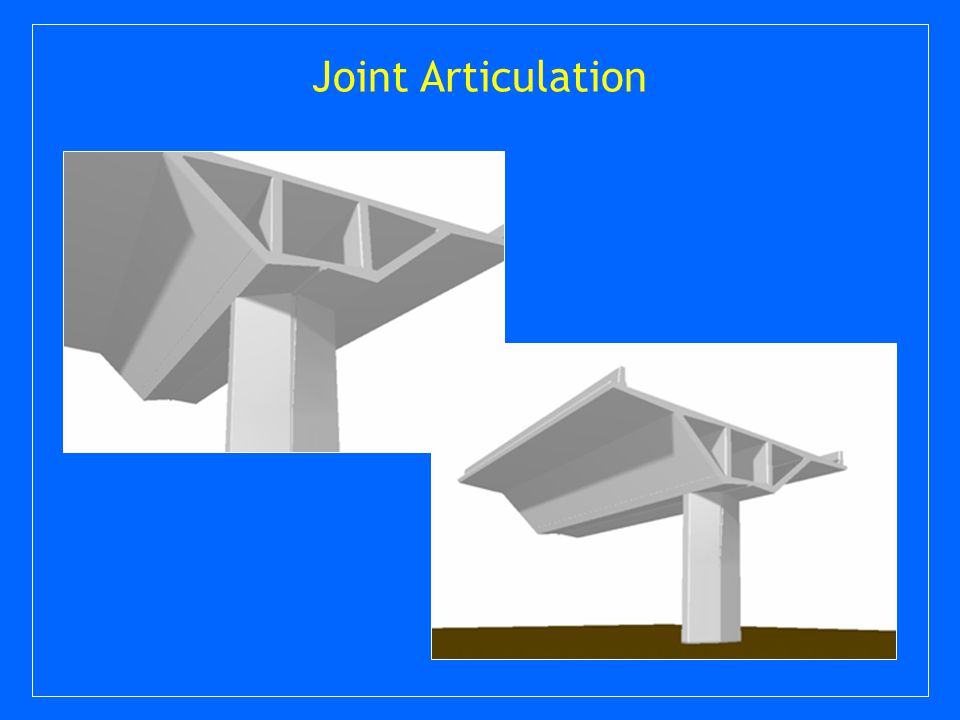The image, rendered in a bright blue, computer-generated style, features a rectangular graphic with a thin white border and a central box. Inside this box, the yellow text "joint articulation" stands out prominently. Two overlapping graphics, positioned in the top left and bottom right corners respectively, depict a detailed architectural joint. Each graphic showcases a white vertical post supporting a horizontal structure reminiscent of a honeycombed bridge section, set against a white background. The top left graphic offers a closer view of the joint, while the bottom right graphic appears zoomed out, revealing a brown floor beneath the post and more of the supporting structure. The overall design emphasizes the structural integrity and connection points in an architectural context.